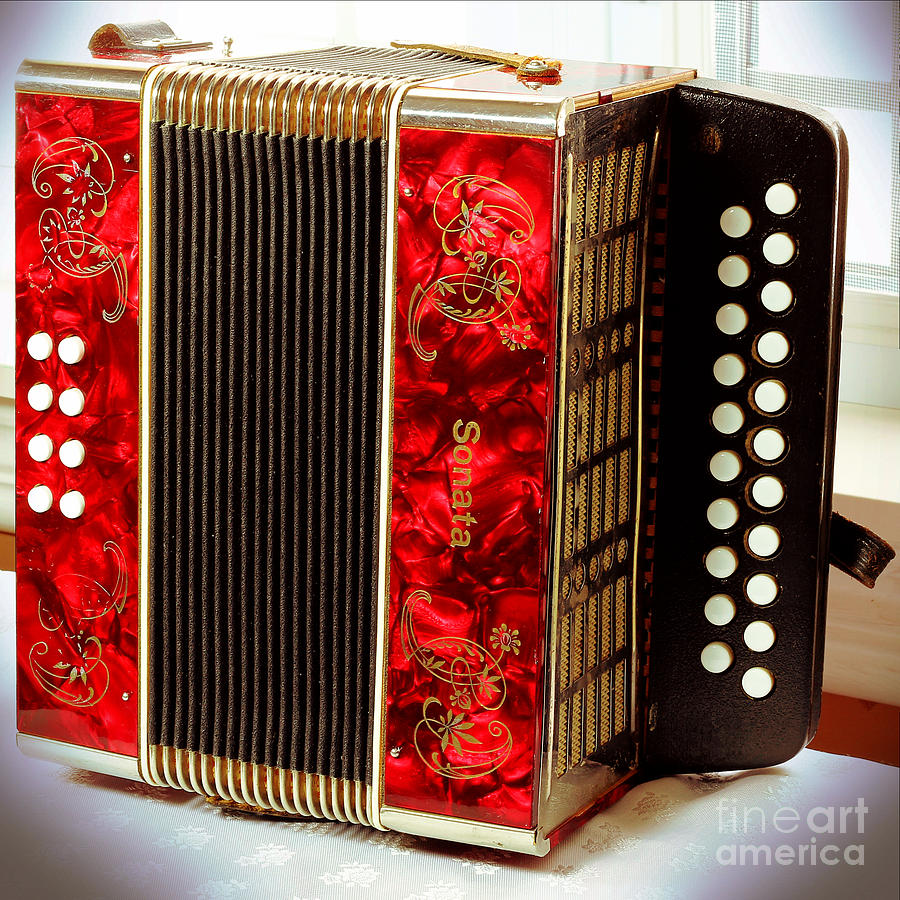This detailed photograph captures a red accordion, characterized by its striking marbled, glassy design and ornate golden filigree scrollwork with leaf and flower motifs. The instrument features compressed black accordion bellows edged in brown, framed by glossy red side panels that prominently display the brand name "Sonata" in gold text. On the left side of the accordion, there are eight white buttons arranged in two rows, set against a black background. The right side showcases a larger button array, possibly twenty white buttons also in rows, adjacent to a black, yellow-hashed speaker grille where sound is produced. A brown leather strap peeks out from the back, used for securing the instrument closed. The accordion is positioned on a white surface, with a subtle glimpse of a wooden floor in the bottom right corner, against a backdrop of white walls and a window. Additionally, the bottom left of the image bears a Fine Art America watermark, marking the photo's artistic provenance.